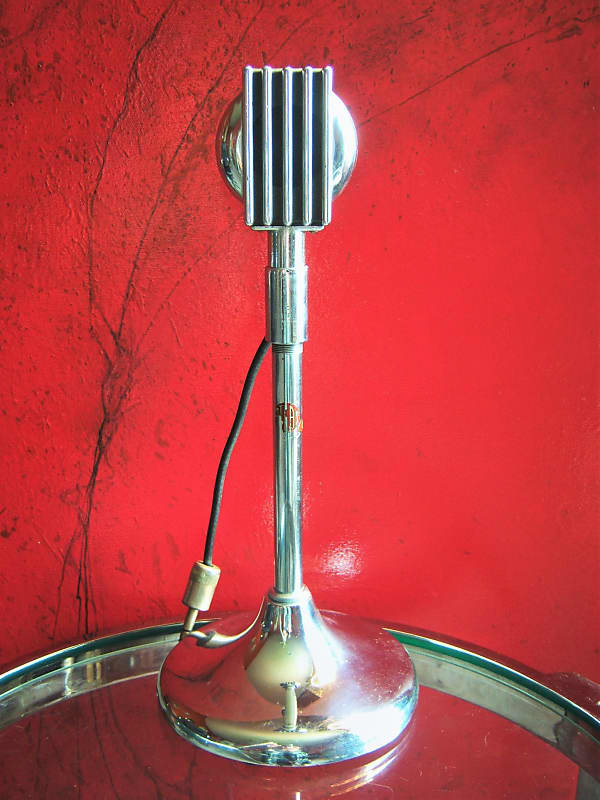The image showcases a vintage-style silver microphone, prominently centered on a round glass table with a metal rim. The microphone's polished stand contrasts slightly with its weathered yet lustrous base. Its design evokes the classic microphones from the late 1930s to 1940s, featuring a series of five evenly spaced vertical pillars and a round metal grille reminiscent of a radiator. A cord is attached to the back of the microphone, reinforcing its operational status. The glass table, reflective and elegant, supports this historical piece against a rich red wall adorned with sporadic black marbling, adding an artistic backdrop to the scene. A small, indistinct red marking on the microphone stand hints at more details, though its specifics remain unreadable. This detailed composition suggests the image could be intended for contexts related to music, recording, or vintage electronics.